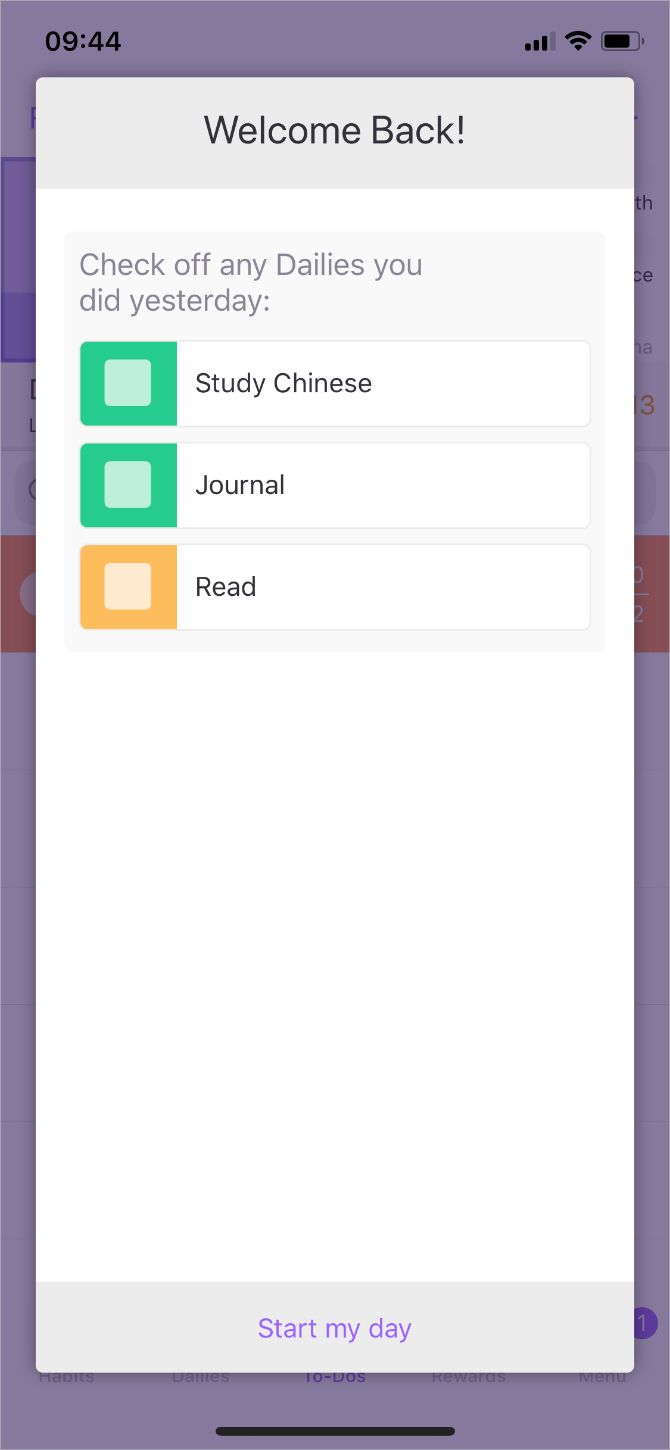This screenshot captures a mobile device's screen at 9:44 AM with nearly full battery and a strong signal. Dominating the screen is a light gray box with black text, welcoming the user back with an enthusiastic "Welcome back!" message followed by "Check off any dailies you did yesterday."

There are three listed activities, each within its own color-coded box. The first box is green and lists "Study Chinese," though it remains unchecked. Similarly, the second green box, labeled "Journal," is also unchecked, leaving ambiguity about whether these tasks were completed. The third box is yellow, marked with "Read," and is likewise unchecked.

At the bottom of the screen, within a gray box, purple text encourages the user to "Start my day." This appears to be part of a daily tracking or habit-forming application.